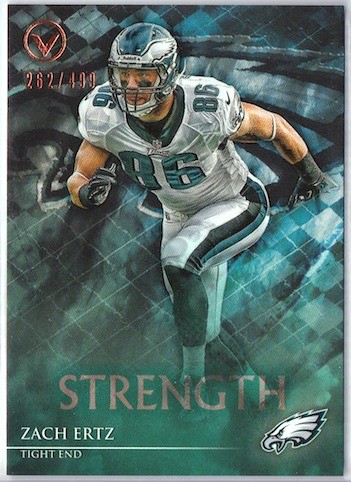The image depicts a detailed football card of Zach Ertz, the tight end for the Philadelphia Eagles, prominently featuring him in a running position. Zach Ertz wears a white uniform with green and black striped pants, complemented by black gloves and a green helmet adorned with an eagle wingspan across the top. His jersey prominently displays the number 86 in green lettering. The card's background is primarily an abstract teal color with square patterns, overlaid with shades of dark blue and white. The Philadelphia Eagles logo, showing the side profile of an eagle's head, is located in the lower right corner, surrounded by a dark border. Above his name, "Strength" is written in light red. On the top left corner, there is a circular logo containing a red V, next to which the card is numbered 262/499, indicating its limited edition status.